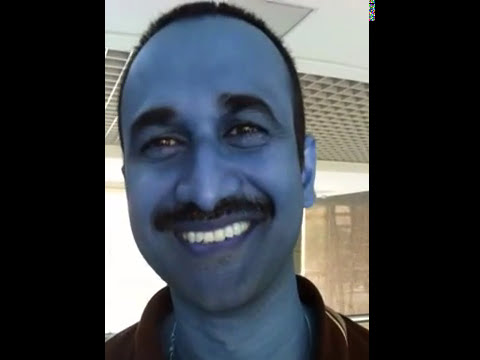The photograph features a man smile directly at the camera, his face and neck dominating the center of the image. His face appears to be tinted a light blue, possibly due to a filter, giving his lips a dark purple hue. He has short black hair, bushy black eyebrows, a black mustache, and is showcasing a big, happy smile with visible, white upper teeth. The man is wearing a collared shirt, which some describe as dark brown, others as red, with a thin necklace that is just barely visible. The background includes white walls and ceiling tiles, a gray AC vent directly above the man, and some patches suggesting a window with a brown curtain. The entire image is framed by two vertical black bars on either side, enhancing the central focus on the man.